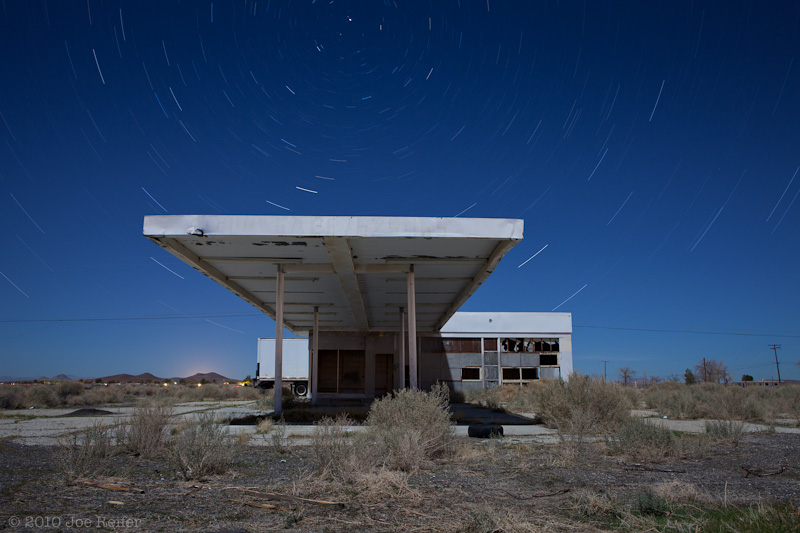This is a detailed photograph of an abandoned service station nestled in an arid, desert-like environment. The old, once-bustling gas station features two garage bays on the right, presumably where cars were serviced, and a cashier or convenience store area to the left. An expansive overhang, supported by light gray poles, stretches out in front where gas pumps would have once operated. The ground is dry and dusty, with patches of tall grass, dead bushes, and tumbleweeds overrunning the area, emphasizing the evident years of neglect. In the distance, a faint mountain range is visible under a network of telephone lines, with a hint of a neighborhood farther back. The sky above is a striking deep blue, dotted with motion trails of stars captured in a mesmerizing circular pattern, indicative of a long exposure or time-lapse photo. Broken glass and the absence of lights beneath the overhang highlight the dilapidated state of the station, painting a vivid picture of abandonment and decay.